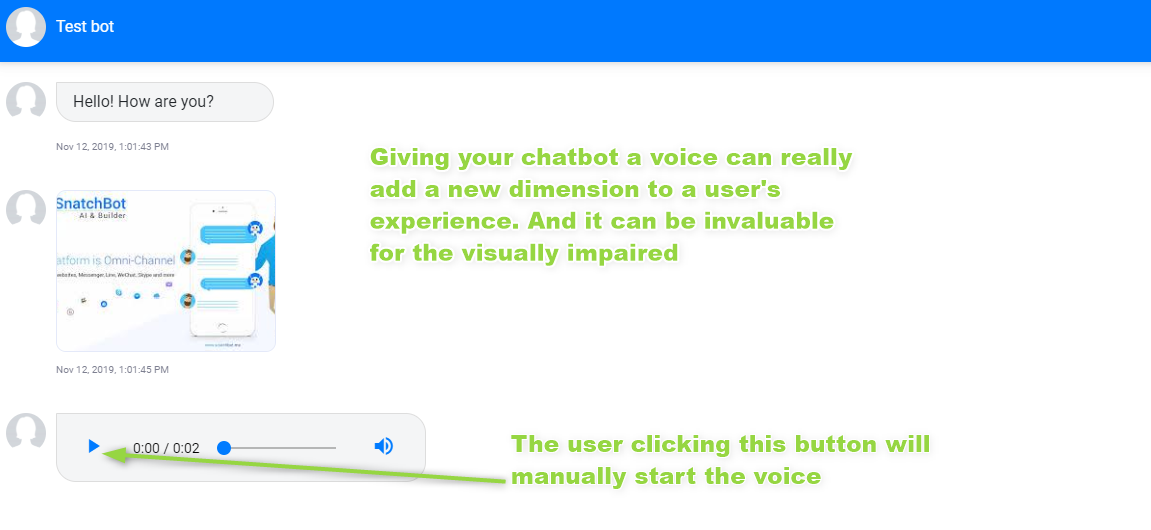At the top of the image is a long, bright blue bar. In the upper left corner, there is an empty profile circle where a user's profile picture would typically appear, but it is currently blank and white. Next to the empty profile circle, the text "test bot" is displayed. Below this section is another white image, accompanied by a gray speech bubble to its right containing the text, "Hello, how are you?" Directly underneath this speech bubble is the date and time: "November 12, 2018, 1:48 p.m."

Further down, there is a box with the word "snatch bot" displayed in blue. Within this box, there is an image depicting a cell phone screen with alternating blue and white speech bubbles. The date "November 12, 2018" is also shown below this screen image.

At the bottom of the image, there is a final gray box. Inside this box, a blue arrow points to a button designed to play and listen to a message. Adjacent to this, a long green arrow extends to the right, accompanied by green text that reads, "The user clicking this button will manually start the voice." Above this, in the same green text, it states, "Giving your chatbot a voice can really add a new dimension to a user's experience, and it can be invaluable for the visually impaired."